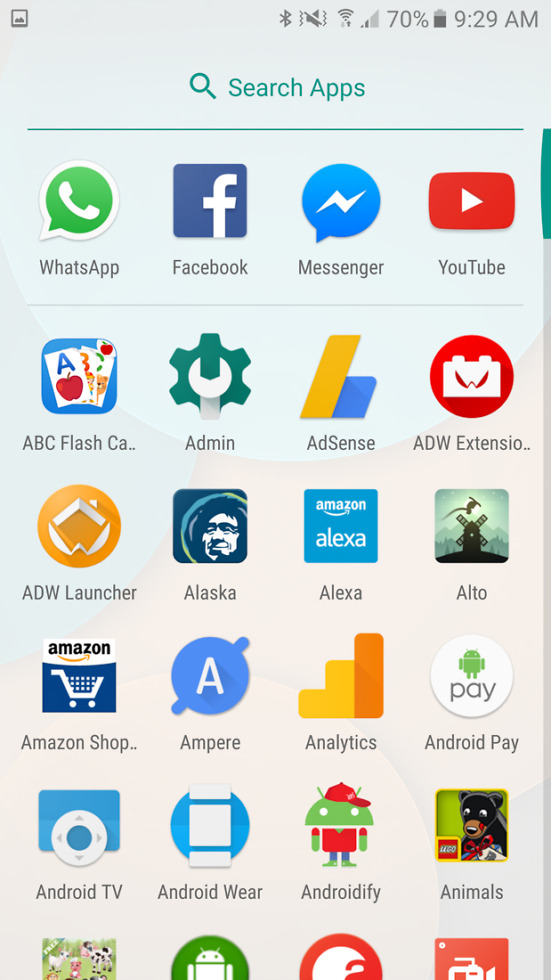A mobile screen displaying a page of various apps. At the top of the screen, there is a search bar accompanied by a magnifying glass icon. Below the search bar, a line separates the search function from the app icons. 

The first row of apps includes WhatsApp with its recognizable green logo featuring a phone icon, Facebook which displays a white "F" in a blue box, and Messenger represented by a blue chat bubble. 

The second row highlights YouTube with its red play button, ABC Flashcards featuring a set of flashcards, and Admin illustrated with a cogwheel icon. AdSense shows a bar graph, ADW Extensions has an image of a brick with a stern face, and ADW Launcher displays a shield with a similar stern face.

On the third row, there is an app labeled "Alaska" with a blue icon featuring a man's face, Alexa represented as a blue square with "Amazon Alexa" on it, and Alto which has an image of a drum jumping over a windmill. There is also Amazon Shop with "Amazon" and a shopping cart, Ampere shows a blue circle with an "A," and Analytics is depicted with a bar chart.

The fourth row includes Android Pay with a white circle stating "Pay" and displaying the Android logo, Android TV showing a controller, and Android Wear represented by white boxes within a blue circle. Androidify features the green Android mascot dressed in a Domino's employee outfit complete with a red hat and polo. Finally, there is an app labeled "Animals" which shows a bear wearing a bow and a small Lego logo at the bottom.